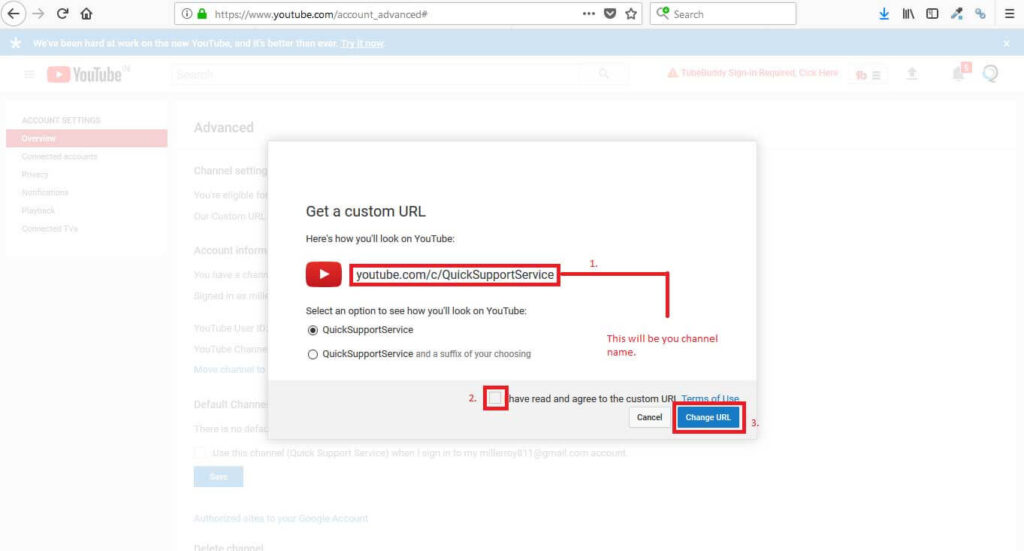The image depicts a YouTube webpage with most elements faded into the background, highlighting a prominent overlay in the center. The overlay reads "Get a Custom URL" with a subheading "Here's how you'll look on YouTube." Beneath this, there is a rectangular box bordered in red, featuring the YouTube logo and a customized URL placeholder that reads "YouTube.com/QuickSupportService." 

A red line extends from the right side of the box, directing attention downward to text that indicates, "This will be your channel name." To the left of this, there is a prompt: "Select an option to see how you'll look on YouTube." Below this are options - the first option, "Quick Support Service," is highlighted in black, while the second, also "Quick Support Service," is not selected.

Centrally located, there is a square checkbox outlined in red with the text, "I have read and agree to Custom URL terms of service." Below this checkbox is a visible blue "Change URL" button with a red border. To its left, there is a "Cancel" button housed within a light gray border. 

In the background, the faded elements reveal a YouTube advanced settings page with the search bar visible at the top, indicating typical HTTPS URL navigation and search functionality.